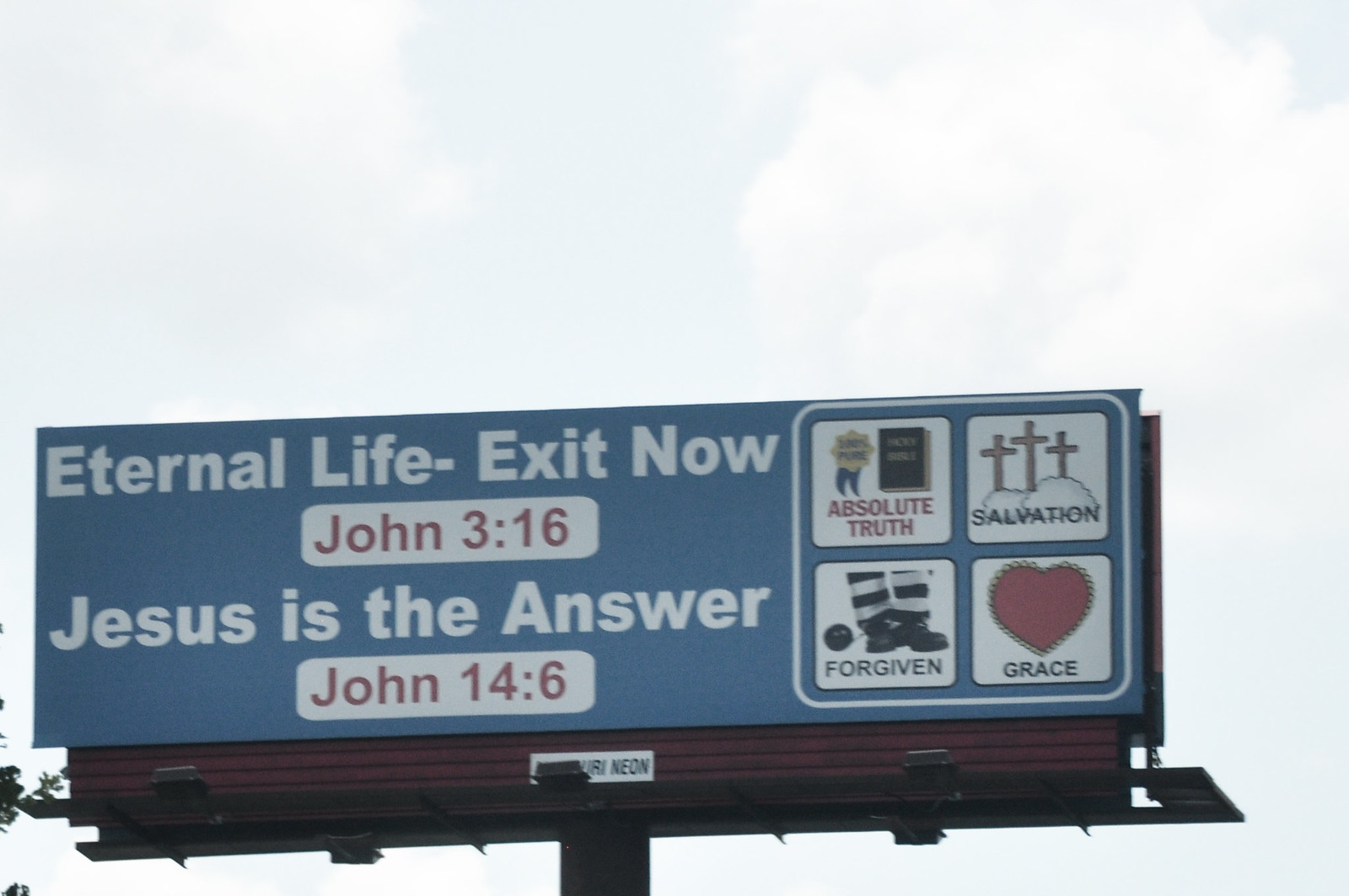The photograph captures a billboard against a pale blue sky dotted with fluffy white clouds. The billboard itself features a medium blue background with prominent white lettering at the top, stating "Eternal Life - Exit Now." Below this phrase, encased in a capsule-like shape with red lettering, is a Bible verse, "John 3:16." Following this, in white letters, it reads "Jesus is the Answer," beneath which another capsule with red lettering displays "John 14:6."

To the right of these inscriptions, there's a square with rounded corners divided into four smaller squares:

- The top-left square reads "Absolute Truth."
- The top-right square says "Salvation" and is accompanied by an image of three crosses.
- The bottom-left square, labeled "Forgiven," includes an indiscernible image.
- The bottom-right square contains a red heart with the word "Grace" beneath it.

The billboard is supported by a black stand, only a small portion of which is visible in the image, emphasizing the billboard itself and the messages it conveys.